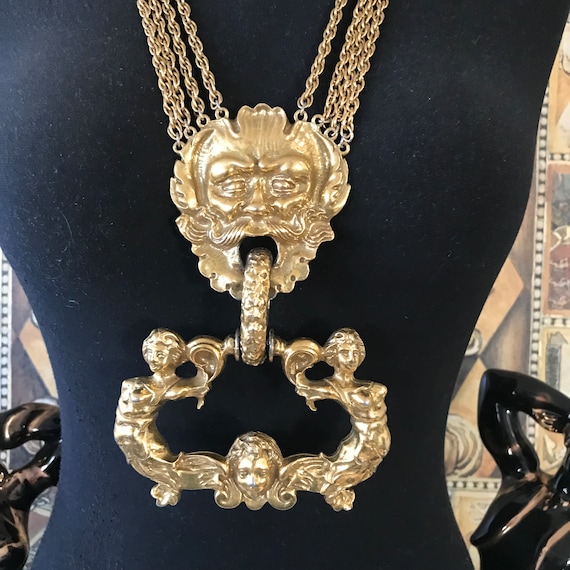The photograph is a detailed close-up of an intricately designed, somewhat gaudy necklace displayed on a black mannequin with a long, narrow torso accentuated by a tight blue shirt. The necklace prominently features four gold chains on each side, descending in an hourglass shape before widening and converging onto a striking gold pendant. This pendant is intricately carved to depict the face of an old man, complete with a mustache and beard, reminiscent of a Green Man, with his mouth open and a hoop emerging from it, resembling a tongue.

Attached to this hoop is a secondary piece resembling a door knocker, where three additional figures are carved: two human-like forms flanking either side and holding onto a central cherubic figure at the bottom. The metal is a light gold, hinting at a possible lesser carat of gold or a gold-like alloy.

The background is adorned with black statues, possibly ceramic and shiny, flanking either side of the mannequin. Behind these statues is a light brown painting, adding depth and contrast to the scene, enhancing the opulence and complexity of the jewelry display.